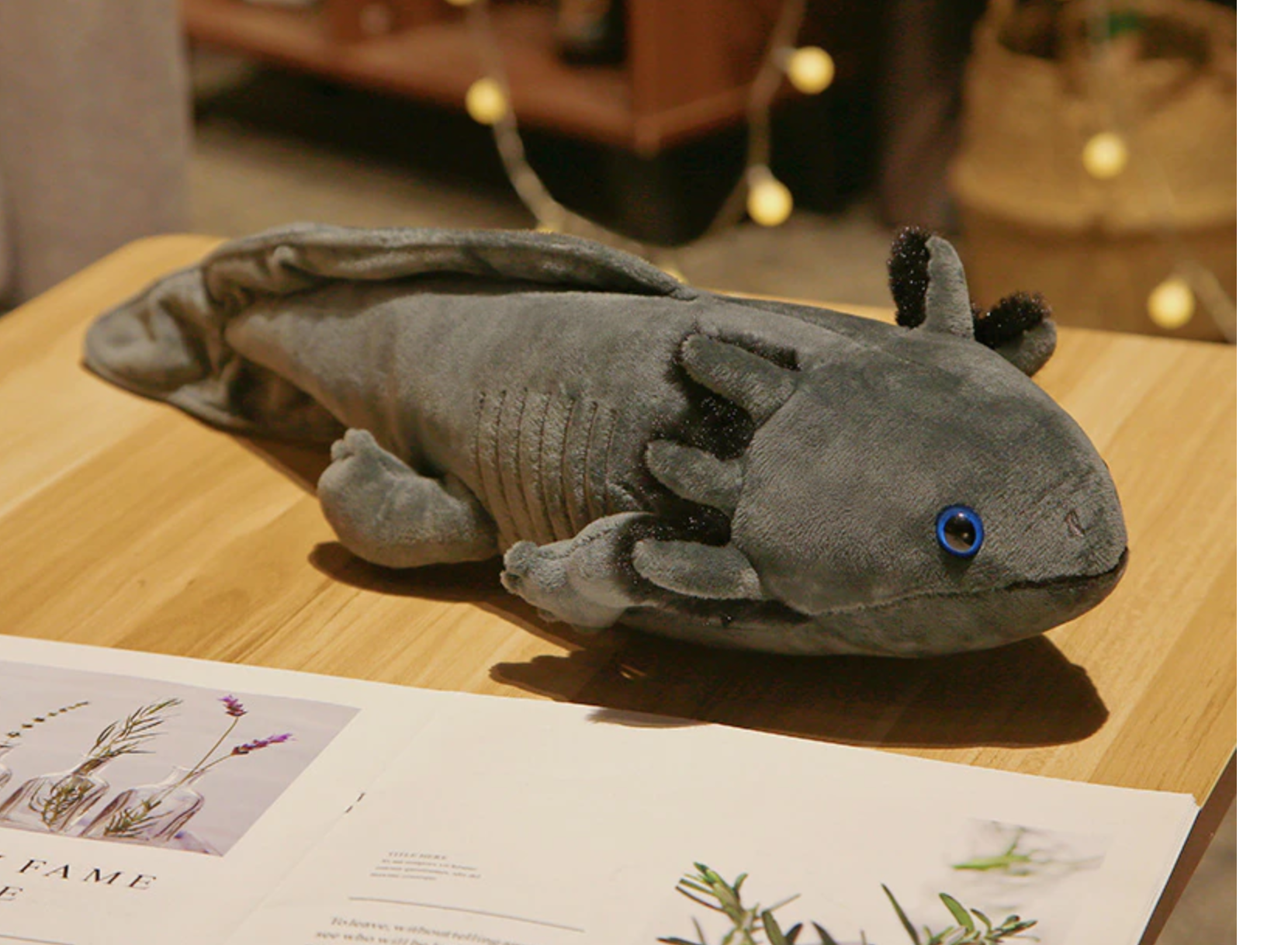The image captures a detailed scene centered on a gray stuffed axolotl sitting atop a light wooden table. The axolotl, a plush toy with distinct black fur adorning the spiky projections on its head, has a singular visible eye that is bright blue with a black pupil. In the foreground, a partially visible paper, possibly a magazine or menu, features a picture of a vase containing purple flowers and the word “FAME” prominently displayed. The background is slightly blurred, revealing a string of hanging lights that add a soft ambiance to the scene, further emphasizing the axolotl as the main focus of the photograph.